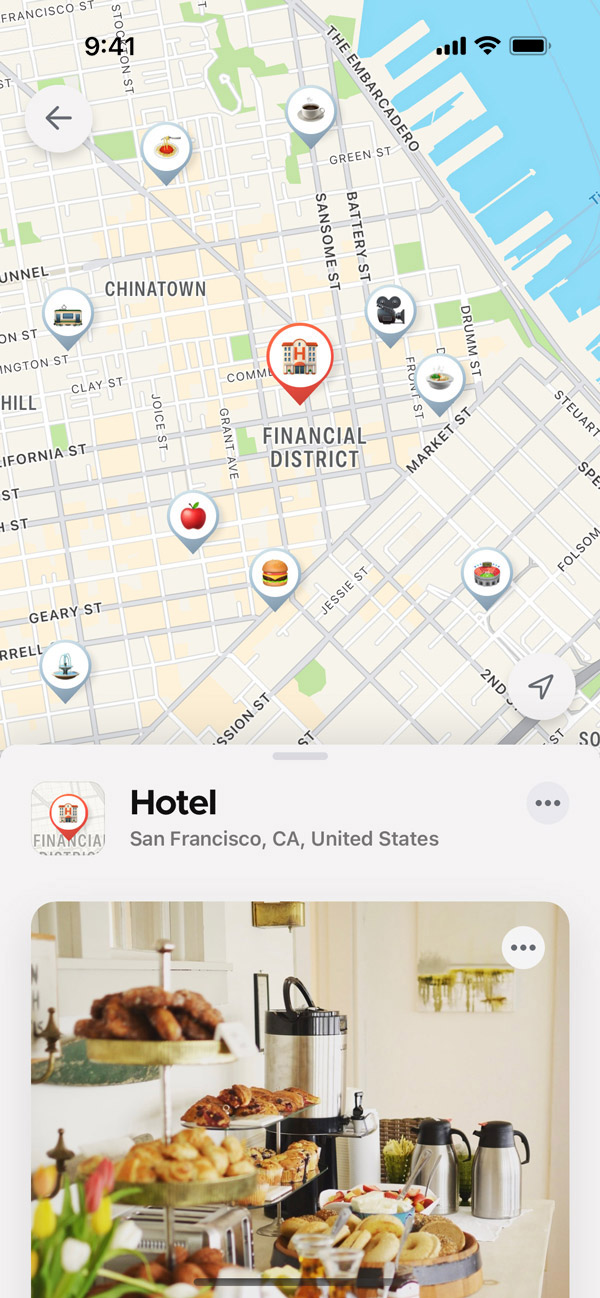The image displays a detailed map interface, possibly from a navigation or city guide application, brimming with icons and layered information. On the top edge, the status bar reveals the device’s connectivity details: full cell phone strength, Wi-Fi signal, and a fully charged battery, listed as 9:41 AM. The primary map interface is set against a creamy yellow backdrop that delineates various city blocks and buildings, while the streets are highlighted in a contrasting off-gray tone.

Various icons pepper the map to signify different points of interest. Red apple icons likely denote grocery stores or markets, brown hamburger icons with tan buns represent eateries or fast food joints, and an old film projector icon possibly indicates a cinema. A prominent feature in the top right quadrant is a large blue body of water, annotated with creamy tan docks extending into it, underscoring the waterfront area.

Significant districts are marked and labeled: the Financial District dominates the map's central area, surrounded by other notable neighborhoods such as Chinatown to its upper left. A pop-up window is positioned towards the bottom, boldly presenting the word "Hotel" in black text. Beneath this, in gray letters, it reads "San Francisco, CA, United States," affirming the city’s location. Depictions of a cozy bed-and-breakfast, replete with a table laden with tan pastries and large black metal coffee pots atop a white cloth, suggest additional accommodation options in the area. This informative and well-illustrated map provides an intricate glance into the bustling landscape of San Francisco, CA.